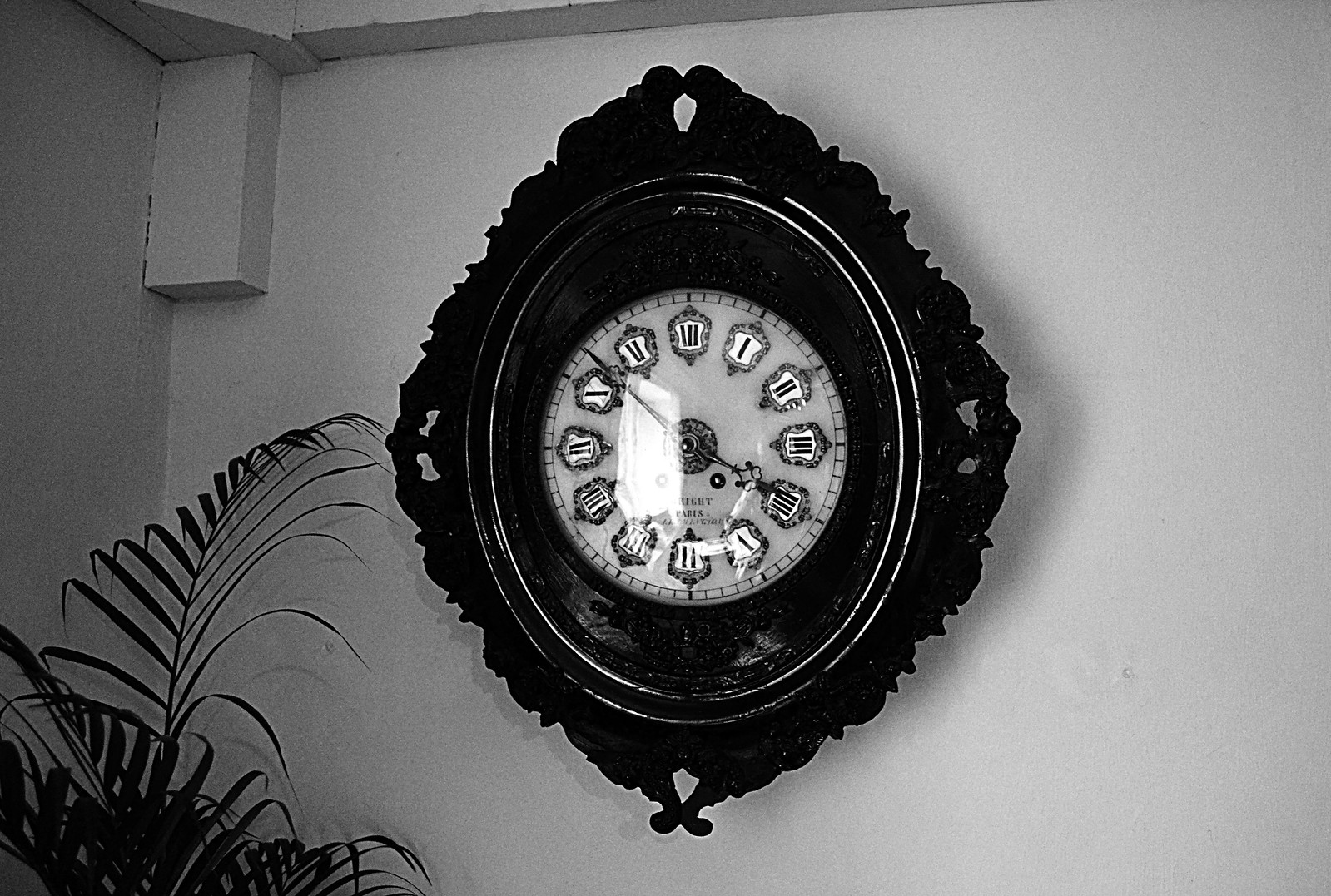This black-and-white photograph captures a corner of an elegantly decorated room. Dominating the center of the image is an elaborate, wall-mounted clock. The clock features a white face adorned with Roman numerals, each encased within intricate, ornate designs. The hands of the clock are also exquisitely detailed, contributing to its overall sophisticated appearance. Surrounding the clock is a large, dark decorative mount that extends outward, enhancing its prominence on the otherwise plain white wall. In the upper left corner of the photo, part of the ceiling is visible, indicating that the clock is hung close to where the wall meets the roof. To the left of the clock, a leafy green indoor plant slightly encroaches into the frame, adding a touch of natural contrast to the scene. While the pot of the plant is not in view, the visible foliage suggests its presence, lending an additional layer of depth to the composition.